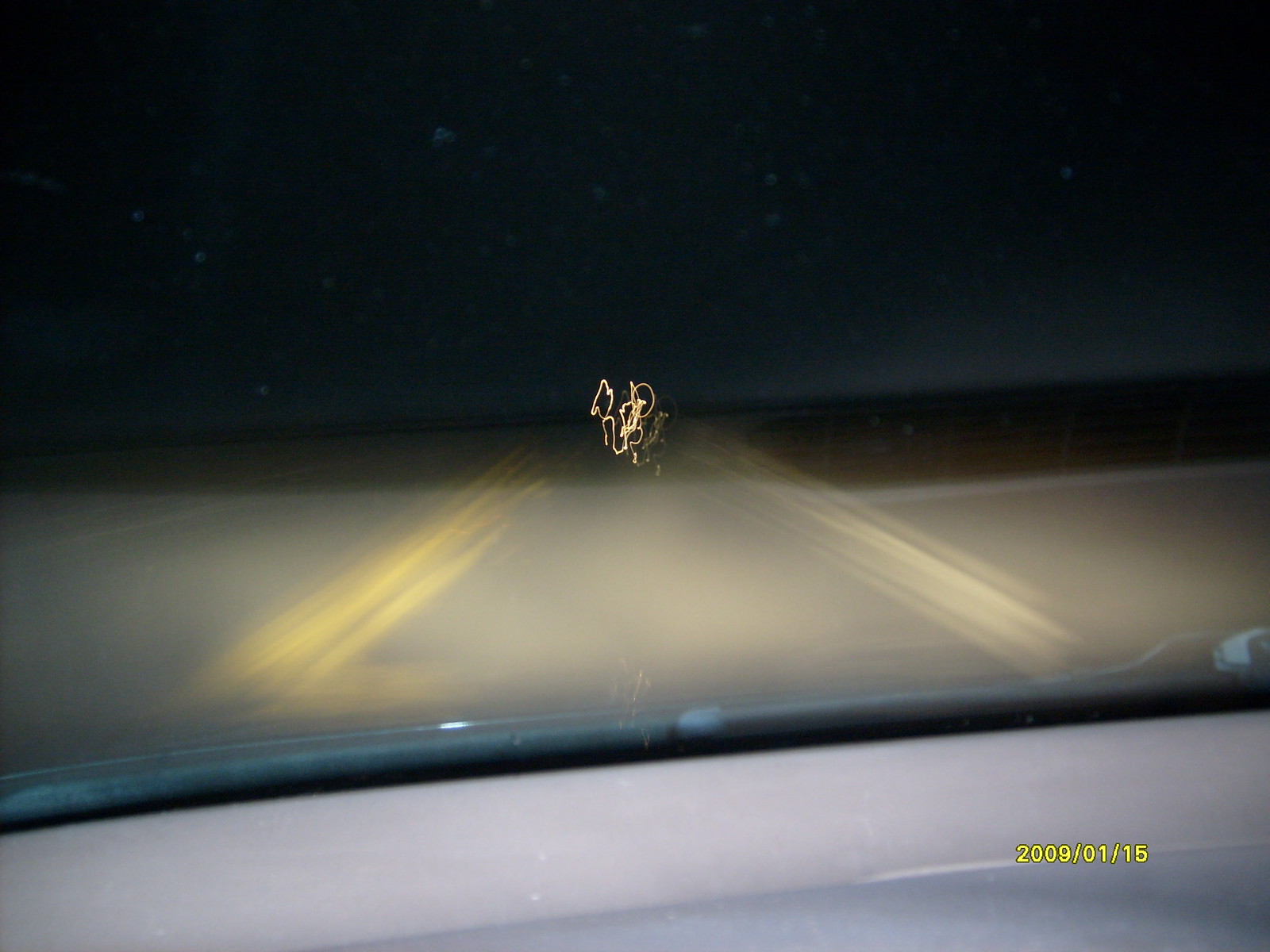This slightly blurry nighttime photograph captures a serene yet slightly disorienting scene. The sky, a deep blue-black canvas peppered with a multitude of twinkling stars, dominates the upper half of the image. The highway below, featuring multiple blurred yellow lines, hints at movement or an extended exposure, giving it a surreal quality. On the right side of the road, a patch of grass is faintly visible. The photo appears to be taken through a car windshield, with the dashboard, a section of the windshield wipers, and the edge of the windshield faintly visible. In the foreground, a squiggly light trail adds an unusual element, likely a result of camera motion during a long exposure. A timestamp at the bottom right corner reads "10-15-2009," marking the exact date this ethereal moment was captured.